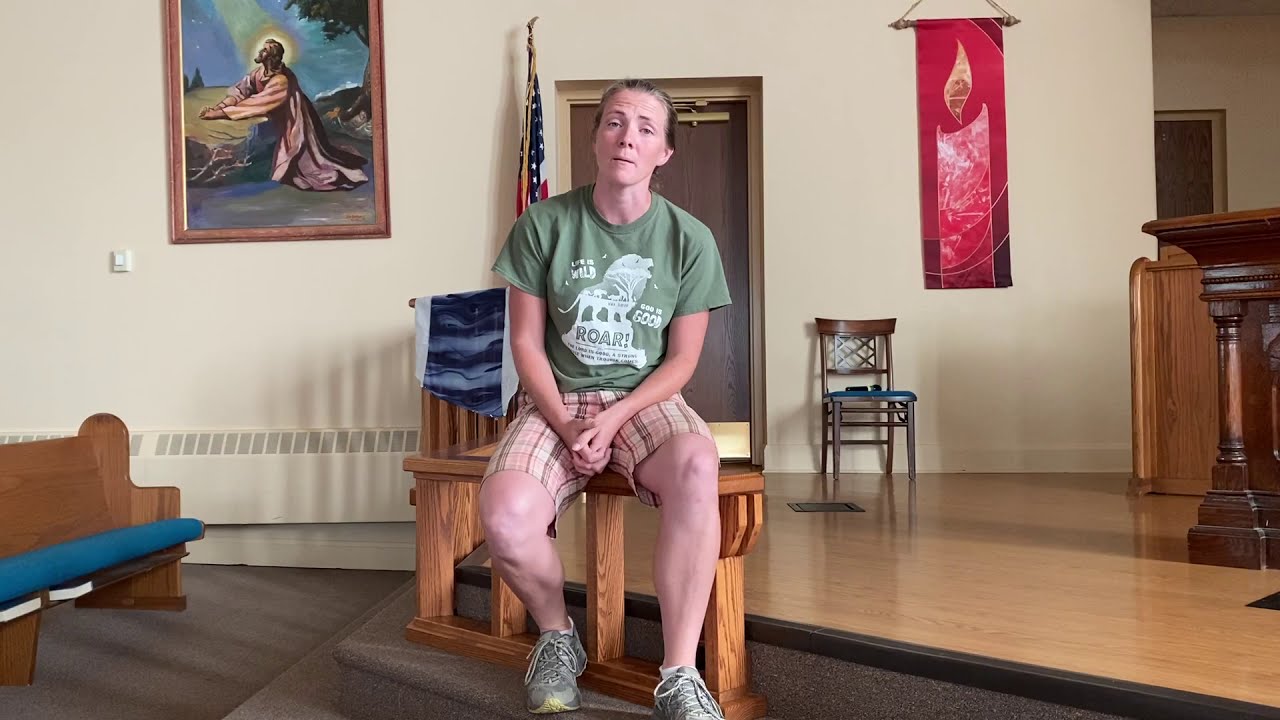The high-quality, color photograph captures an indoor scene of a chapel or church, taken during the middle of the day. The image is in landscape orientation, with the main subject, an older woman with almost gray hair, situated prominently at the center. She is seated on a wooden bench covered with a blue cushion, positioned at the edge of a staircase leading up to a wooden altar on the right.

The setting around her is detailed and well-lit, featuring white walls adorned with various pieces of artwork. To the woman's left, a pew is visible, and above it hangs a painting depicting Jesus kneeling in prayer at a rock. Behind her, a brown door can be seen, along with an American flag. To her right, there is a vertical banner with a red candle design hanging near the pulpit area.

The woman is wearing a green t-shirt with the word "Roar" emblazoned on the front, plaid shorts in shades of tan, red, and black, and gray athletic shoes that appear worn. Her knees are exposed, showcasing a mix of muscular feet and skinny arms, suggesting she is an older woman. The setting, combined with the detailed depiction of the woman's clothing and features, conveys a serene and reverent atmosphere within the religious space.